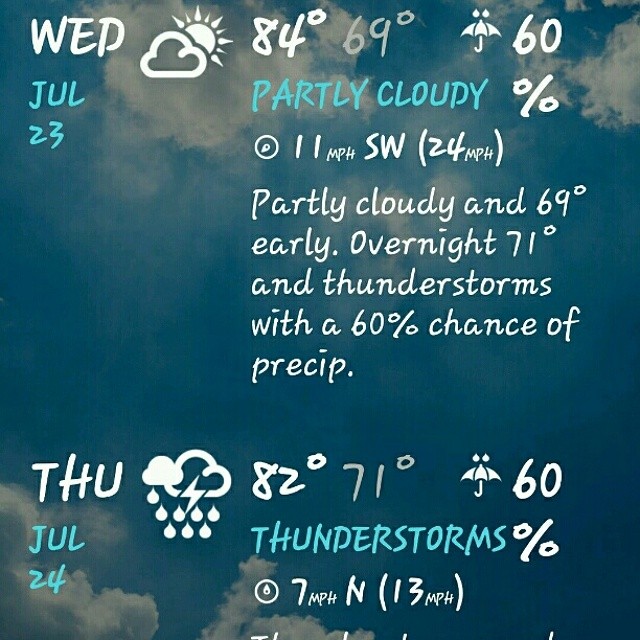The image is a detailed weather forecast advertisement set against a light to deep blue sky backdrop with white clouds dispersed throughout the top and bottom of the scene. In the upper left corner, "Wednesday" is displayed in white text. Adjacent to it, there is an emblem featuring a cloud and a sun, followed by the temperatures, "84°F" and "69°F." Below, icons of an umbrella with raindrops accompany a "60%" chance of precipitation. The forecast specifies that July 23rd will be partly cloudy with 11 mph southwest winds, gusting up to 24 mph. Early in the day, it will be 69°F, and overnight temperatures will be around 71°F with a chance of thunderstorms and a 60% likelihood of rain.

In the bottom left corner, "THU" for Thursday, July 24th, is highlighted, followed by weather icons depicting a filled white cloud next to an outline of a cloud with a lightning bolt and raindrops. The day's high will be 82°F and the low will be 71°F. There is a 60% chance of thunderstorms accompanied by north winds at 7 mph, with gusts up to 13 mph.